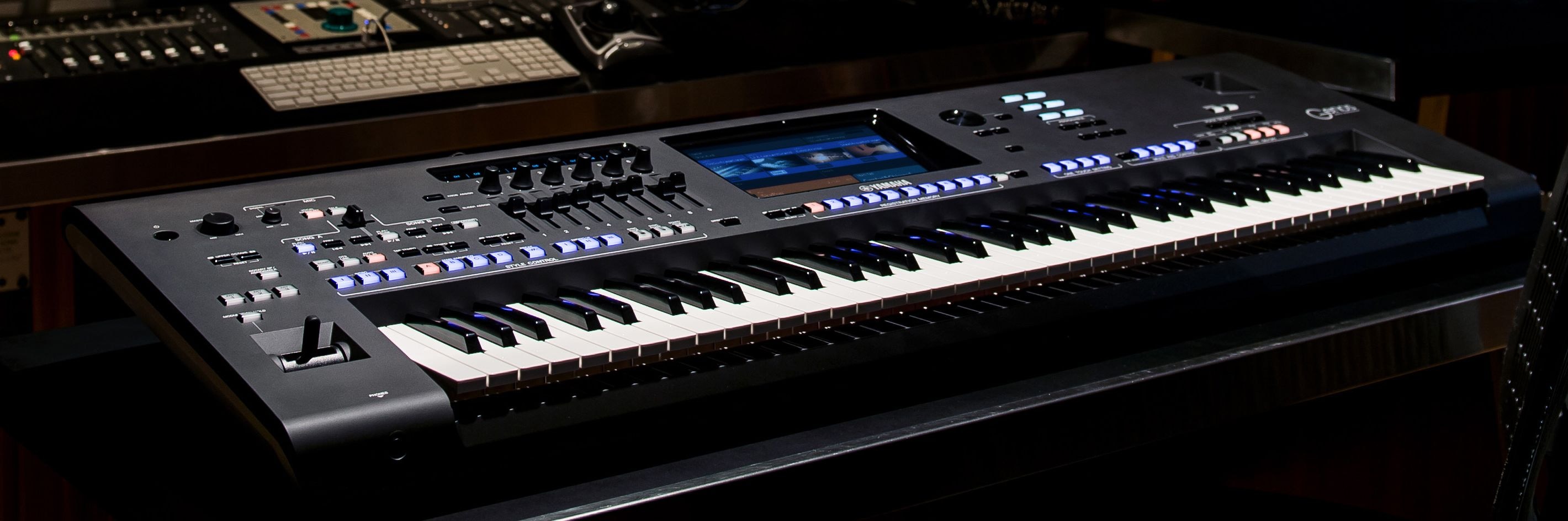This color photograph showcases a professional-grade Yamaha keyboard situated as the centerpiece of an expensive, high-tech music studio. The large keyboard, adorned with an array of buttons, sliders, knobs, and switches, dominates the frame from the bottom left to the top right, with the black and white keys facing right. A digital screen is centrally positioned at the top of the keyboard, bearing the Yamaha logo beneath it. The dimly lit studio is illuminated primarily by the keyboard itself, revealing additional musical and computer equipment in the background, including what appears to be an Apple or Bluetooth keyboard and various other electronic devices. The image is taken from an angle that suggests the photographer is standing above or in front of the keyboard, emphasizing the sophisticated and professional environment of the music studio. Colors noted in the scene include shades of blue, light pink, black, and white.